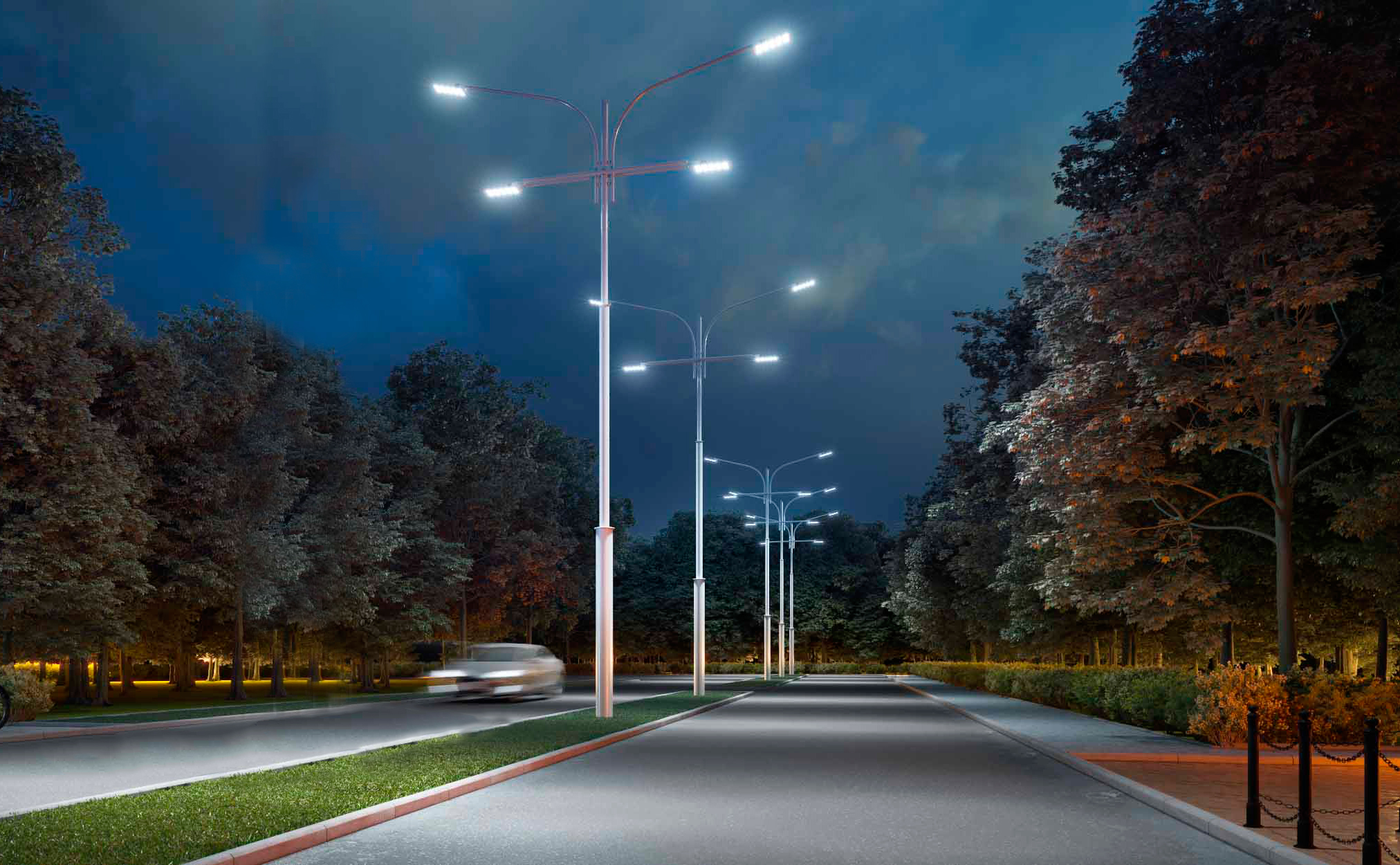The image is a conceptual 3D rendering or a long exposure photograph taken at night or possibly just after dusk. It showcases a city street with a blacktop road divided into two lanes. The central feature is a small grassy island, bordered by a concrete curb, positioned between the lanes. Tall streetlights, designed in a unique 'T' shape with bright LED lights at their tips, illuminate the area. These streetlights appear along the grassy median and at intervals down the street.

On the left lane, a white car is captured in motion as a complete blur, conveying a sense of speed. The right side of the street features a sidewalk lined with bushes and metal poles connected by chains. Alongside the road on the left side, there's a row of trees with lush green leaves, underlit by an amber glow, enhancing the nighttime ambiance. The sky is a dark blue, enhanced by thick clouds touched with subtle golden hues, possibly illuminated by the remnants of a setting sun.